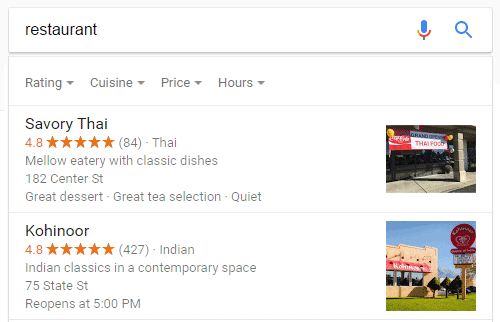The image depicts search results from a Google query for restaurants. The first result that appears is for "Savory Thai," which boasts a remarkable 4.8-star rating. This establishment is described as a mellow eatery offering classic Thai dishes. It is praised for its great desserts, excellent tea selection, and quiet ambiance. The second result is for "Kohinoor," which also has an impressive 4.8-star rating. Kohinoor specializes in Indian classics served in a contemporary setting, and it opens at 5 PM.